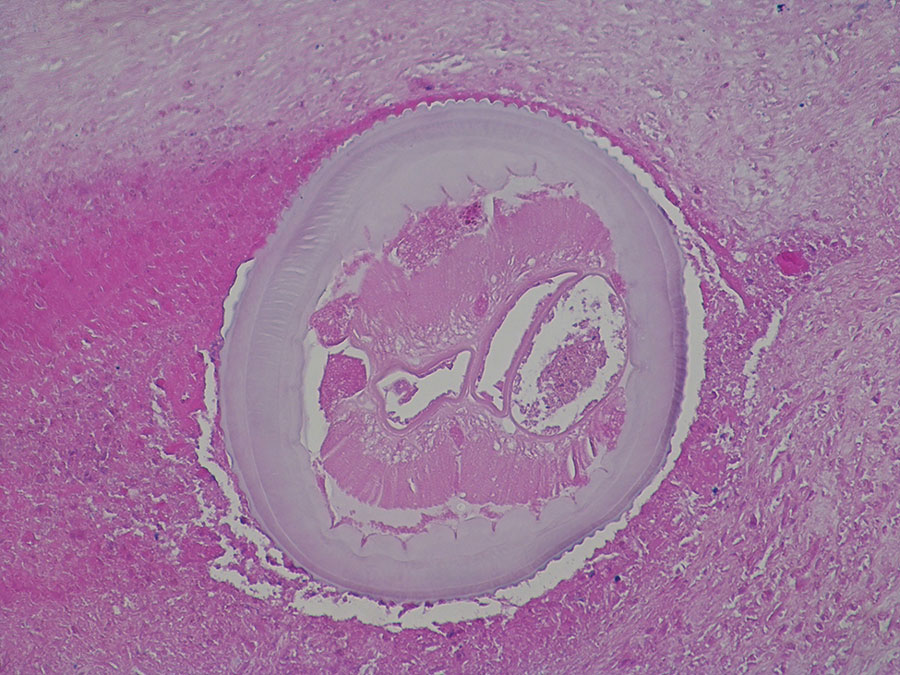This image appears to be a stained microscopic photograph of a cell on a slide, dominated by various shades of purple ranging from very light to dark, with some off-white elements. Centrally, a large, roughly circular shape, light purple in color, features a darker purple nucleus that occupies most of the space. Surrounding this central figure, the frame is filled with irregularly shaped, possibly white organelles and a complex pattern of darker purple hues. There are additional details, like pinkish tones and gray borders, where the central mass contains smaller structures and some spike-like protrusions. This intricate and textured background enhances the depth and complexity of the visual field, suggesting a highly detailed biological specimen under microscopic examination.